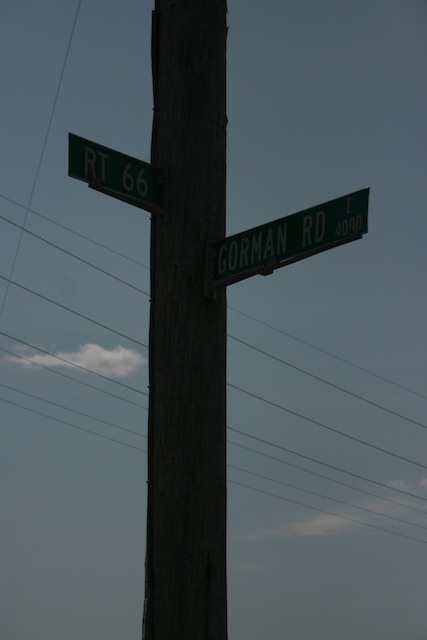The photograph captures a shadowy outdoor scene featuring a wooden pole adorned with street signs. The sky in the background is a dimly lit bluish gray, with only a couple of wispy white clouds scattered across it. Horizontal telephone wires criss-cross behind the pole, running slightly diagonally from the upper left to the lower right. There are two rectangular street signs affixed at right angles to the vertical pole. Despite the low light conditions making it challenging to read the exact text, it is discernible that the first sign on the left-hand side, likely indicating Route 66, has white text on a green background. The sign on the right-hand side possibly reads Conway Road or Gorman Road, also featuring white text on a green background, with some additional numbers too dim to make out. The wooden pole stretches the entire height of the image, from the bottom to the top, set against the dusky sky.